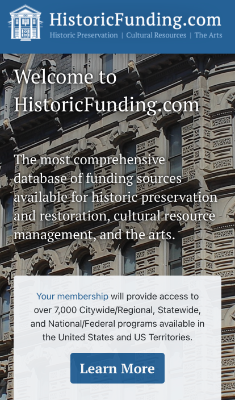**Caption:**

Discover the Ultimate Resource for Historic Funding

This online advertisement for HistoricFunding.com introduces a comprehensive database designed to support historic preservation and restoration, cultural resource management, and the arts. The ad features a striking black-and-white image of a historic brick or cinderblock building, overlaid with a white and blue banner. The banner prominently displays an iconic house emblem, symbolizing historic architecture.

Text within the ad welcomes users to HistoricFunding.com, describing it as the most extensive database of funding sources available. The information highlights that membership grants access to over 7,000 programs at the citywide, regional, statewide, and national levels throughout the United States and its territories. A call-to-action is present, encouraging users to "Click to Learn More."

This visually appealing and informative advertisement aims to guide individuals and organizations seeking financial support for their historic and cultural projects.